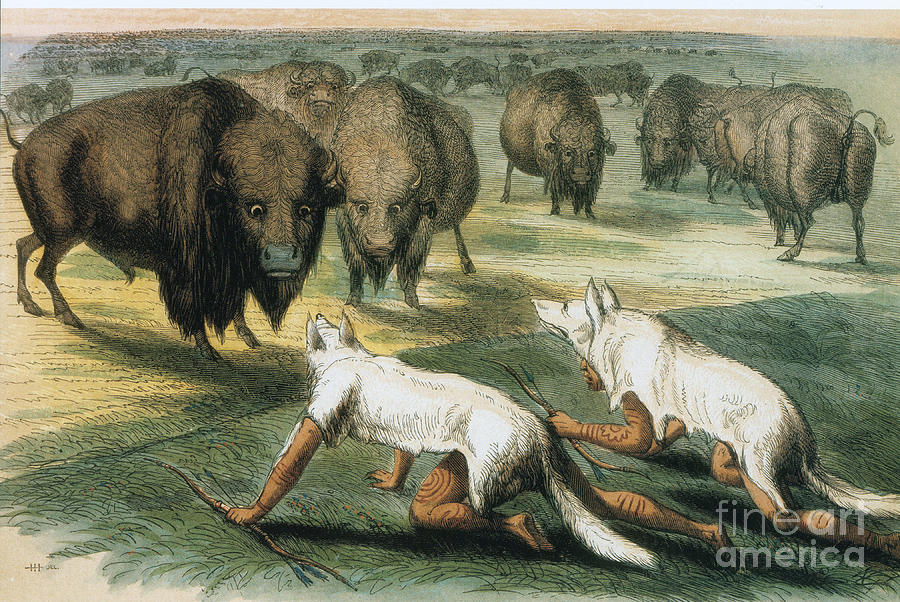The image is a detailed color illustration in landscape orientation, showing a dramatic scene of two men disguised as white wolves stealthily approaching a herd of bison. The men, dressed in white wolf pelts that cover their heads and bodies—with muzzles, ears, and tails included—are crawling on all fours through dark green grass. Their arms and legs are marked with tattoos and they carry spears in their hands. 

In the background, a group of bison is arranged side-by-side across the top half of the image, standing in a grassy pasture that stretches to the horizon. Some of the bison are gazing down suspiciously at the men, their expressions ranging from alert to curious. The bison vary in color from dark brown to lighter brown, adding depth to the illustration. The illustration style uses close hash marks and washes of color to create a textured, painterly effect.

In the lower right corner, a white watermark reads "Fine Art America." This cleverly crafted image blends traditional art techniques with a contemporary composition to depict an intense, almost surreal moment between the hunters and their prey.